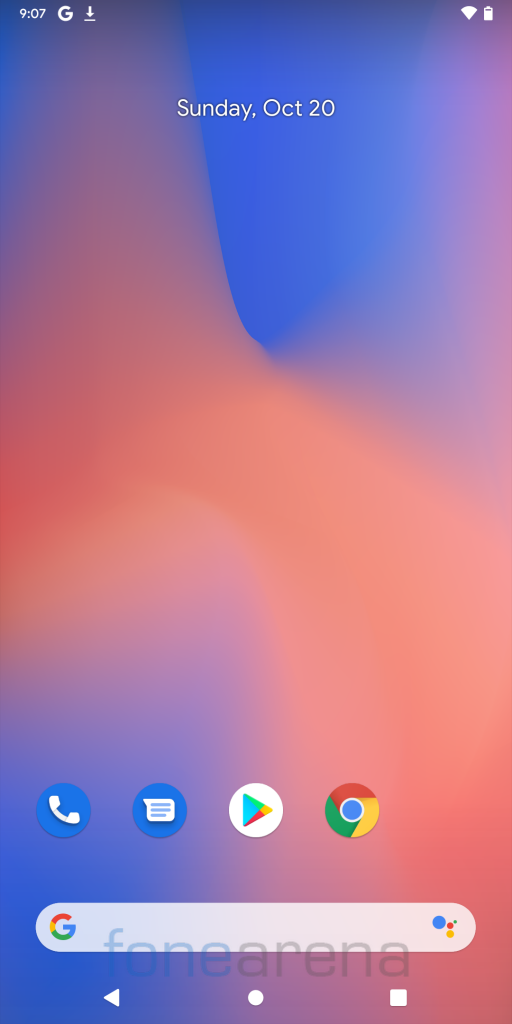The image showcases a colorful smartphone home screen with a vibrant blue, red, and pink wallpaper. At the top, a status bar displays various icons. On the top left, the current time reads 9:07, followed by a white Google icon represented by a "G," and a download icon depicted as an arrow pointing downwards to a line. On the top right, the battery status and Wi-Fi signal icons are positioned, both also in white.

Centrally placed below the status bar is the date, displayed in white text: "Sunday, October 20."

At the bottom of the screen, a row of app icons is neatly arranged. From left to right, the icons include:
- A blue and white calls icon.
- A blue and white messages icon.
- A Google Play Store icon characterized by a white background with a multicolored play button in blue, green, yellow, and red.
- A Chrome browser icon, consisting of a circular design with blue, red, green, and yellow segments.
- A Google search bar featuring a white background, a multicolored "G" (red, yellow, green, and blue), and an Assistant icon represented by four colored circles (blue, orange, red, green, and yellow).

Directly beneath the Google search bar, the text "Phone Arena" is displayed, with "Phone" written in blue and "Arena" in grey. Additionally, navigation icons in the form of a triangle, circle, and square can be seen, representing common smartphone interface elements.